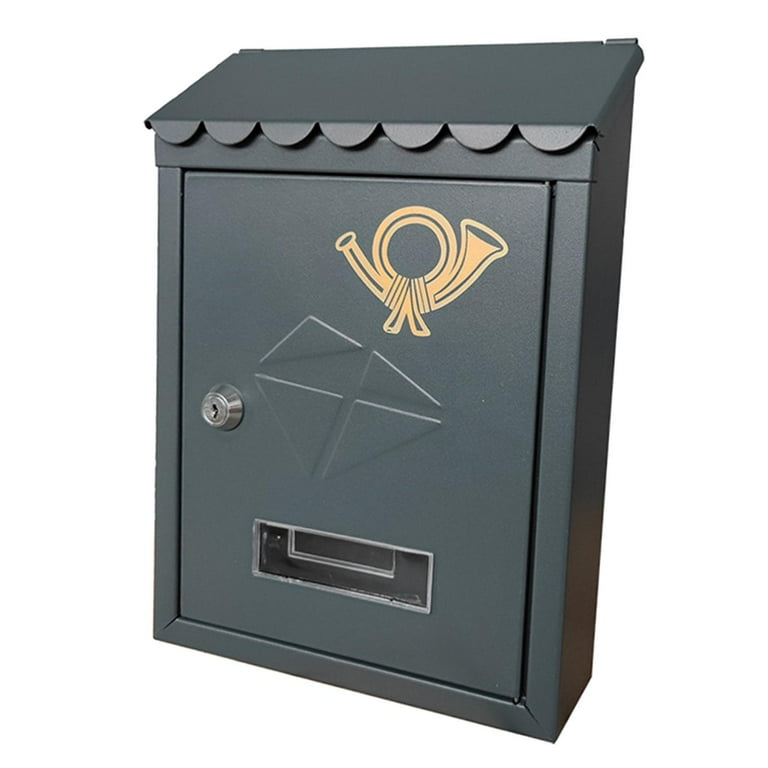The image depicts a large, deep green metal mailbox designed for the exterior of a home. It features a key lock on the front to secure the mail once it is deposited through a lid that lifts up. There is a small window at the bottom of the front door, allowing you to see if there is mail inside. Additionally, the mailbox has a distinctive gold Bugle logo in the upper right corner of the lockable door. The front of the box also includes a black and silver panel, possibly for added design or function. The overall design includes curtain-like decorations on the lid, further enhancing its aesthetic appeal.